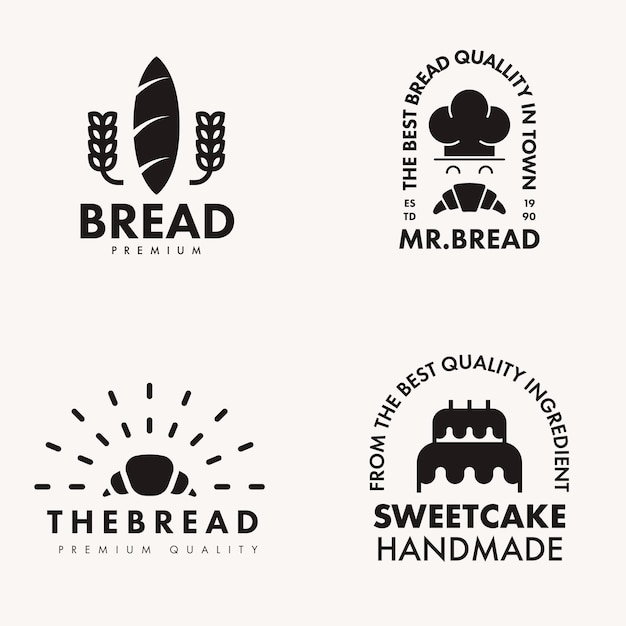This image features four black and white vector graphics of potential bakery logos, each occupying a quadrant of a single layout. The top-left logo showcases a vertical loaf of bread flanked by wheat stalks on either side, with the words "BREAD PREMIUM" written beneath it. The top-right logo displays a whimsical design of a chef’s hat with cartoonish eyes and a croissant acting as a mustache, accompanied by the text "MR. BREAD" below and the phrase "THE BEST BREAD QUALITY IN TOWN" encircling it. The bottom-left logo highlights a croissant with sun rays emanating from it, subtitled with "THE BREAD" and "PREMIUM QUALITY." Lastly, the bottom-right logo features an illustrated layered cake topped with three candles and bears the text "SWEET CAKE HANDMADE," with "FROM THE BEST QUALITY INGREDIENT" arched around it. These designs are likely part of a mockup or template intended for bakery branding options.